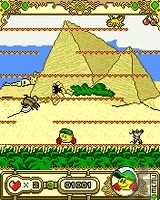The screenshot appears to be from a video game. At the top of the image, there's a decorative gilding in a tan color featuring small green dots. Below this gilding, a goldish insect, possibly a bee, is depicted along a line. The background transitions from a white sky in the upper section to a blue sky beneath it.

Prominently, the scene includes two Egyptian-style pyramids: the larger one on the left is slightly tilted, while the smaller one stands to the right. Both pyramids are a tan color. In the foreground, green bushes can be seen, along with a small hut situated to the left and a noticeably oversized bee hovering nearby.

Below this section, the terrain changes to sand with another horizontal line. Here, a yellow creature's head, adorned with a green hat and a red top, is visible. Following this motif, there’s a sequence of tan and green bushy lines.

In the bottom panel, there's a heart symbol next to an 'X' and a set of numbers that possibly read "05001." Additionally, there's a circular icon featuring the yellow creature's head again, this time including two red hands, and the creature is wearing the same green baseball cap.